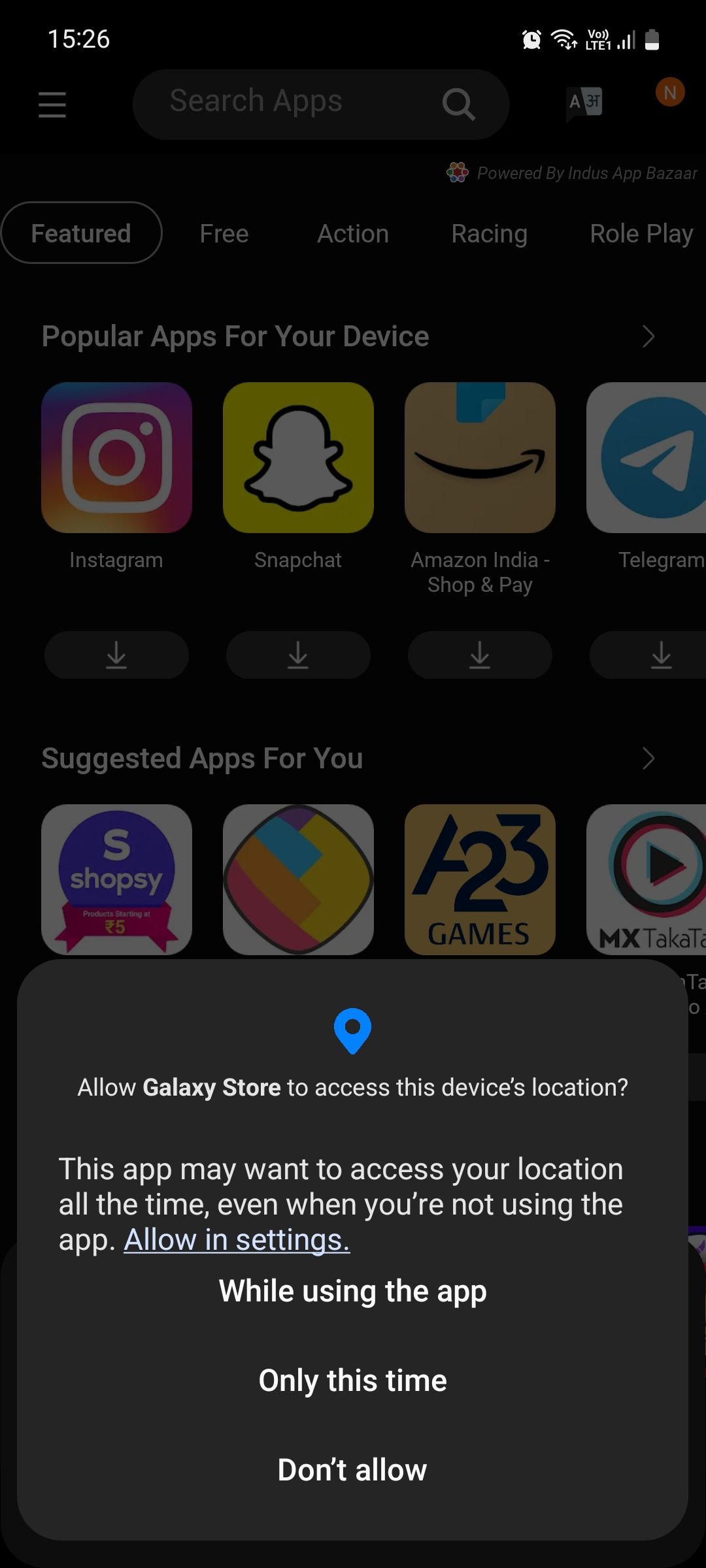This is a detailed screenshot from a smartphone, showcasing various on-screen elements. At the top of the image, the time is displayed in military format as 15:26, accompanied by a clock icon. To the right of the time, there is a Wi-Fi symbol indicating a strong connection with two arrows, one pointing down and the other up, suggesting data is being transmitted both ways. Next to it, the text "LTE" signifies the type of network connectivity. A signal strength bar appears next, showing three out of four bars filled, indicating good signal strength. The battery icon shows a quarter charge remaining.

Dominating the screen is a system prompt with a location icon, querying, "Allow Galaxy Store to access this device's location?" The prompt warns that the app may want continuous access to location data, even when the app is not in use. Below this message are three interactive options: "Allow and settings" (underlined), "While using the app," "Only this time," and "Don't allow."

In the background, partially visible at the top, is a navigation bar featuring a hamburger icon (three horizontal lines) and a search field labeled "Search apps" where users can type queries. A magnifying glass icon and a microphone icon for voice search flank the search bar. Below, there's a section highlighting app categories such as "Featured," "Free," "Action," "Racing," and "Role Play," with "Featured" being highlighted. Further down, two rows of social media app icons, four per row, are visible, though somewhat obscured by the overlaid prompt.